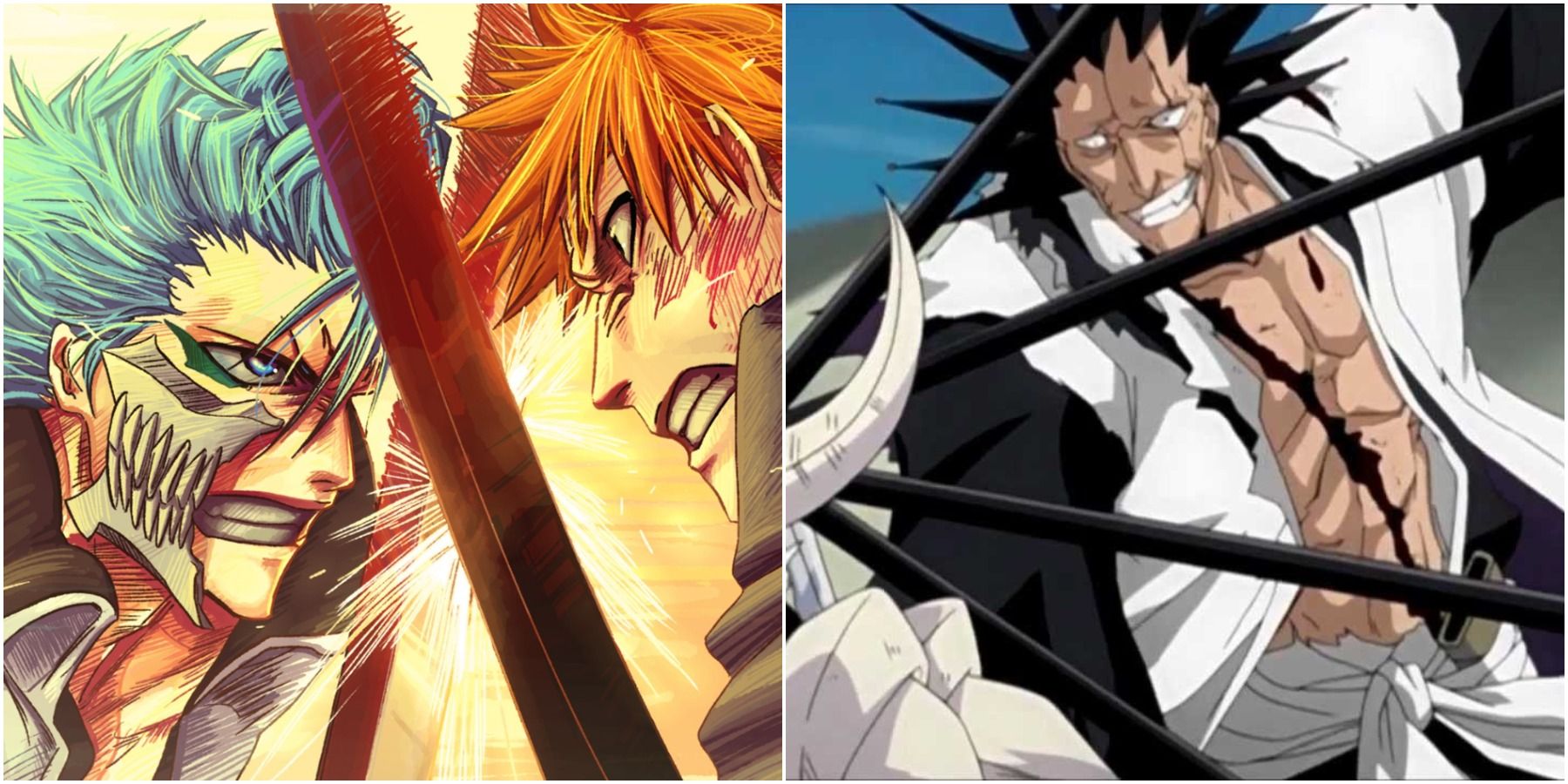The image is a composite of two illustrations from the anime Bleach, separated by a thin white line. On the left illustration, two characters are fiercely clashing their swords, generating visible sparks. The character on the left has spiky sky blue hair, blue eyes, a skeletal mask covering the right side of his face, and a high black collar trimmed with white. Opposite him, the main character with spiky orange hair stares him down, their intense expressions emphasizing the heated battle. The right-hand illustration features another spiky-haired man, this time with black hair. He has a distinct scar running over one of his eyes and another scar down his chest, visible through his open black and white shirt. He is surrounded by mysterious black poles and a white spike, appearing poised to engage in combat.